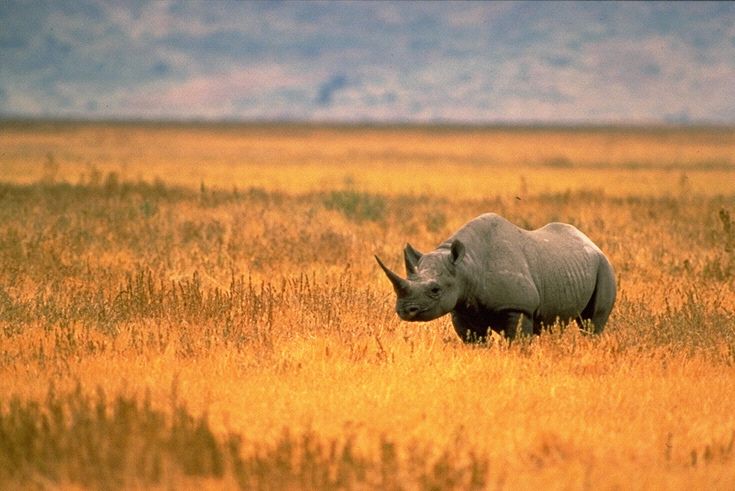The photograph captures a solitary rhinoceros standing sternly in a wilderness, possibly in Africa, amidst a field of tall, brownish-yellow and orange grasses. The rhino, a dark gray figure and central focus of the image, is positioned slightly to the right but facing directly toward the camera, appearing almost as if it's gazing at the viewer. Surrounding the rhino, the tall grasses blend into blurred hues of green, yellow, and orange, creating a striking contrast against the sharp, detailed presence of the rhinoceros. The backdrop of the photograph is a wide, open expanse devoid of trees, extending to a blurred horizon. Above, a subtly dark blue sky, tinged with clouds and hints of yellow and red, suggests the onset of evening, further enhancing the serene yet solitary atmosphere of the scene.